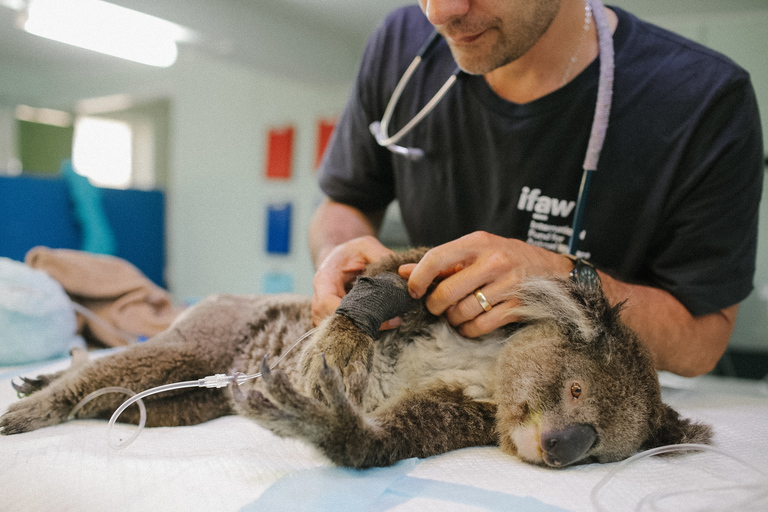The image captures a detailed scene in a veterinary clinic, specifically depicting a koala bear undergoing medical treatment. The koala bear lies sedated on an examination table, its brown eyes open but calm. The animal is positioned on its side with an IV tube taped to its forearm using black cotton tape. A dark blue-shirted man with a white IFAW logo on his chest, a stethoscope around his neck, and a black stubble beard examines the koala’s injured arm. The individual, visible only from the nose down, also wears a silver neck chain and a ring on his ring finger. The setting features white walls, fluorescent tube lighting, and various colored charts and files in the background, indicating an organized emergency or examination room. The photograph, taken in landscape orientation, is a clear example of photographic representationalism realism, capturing both the urgency and care in veterinary medical practice.